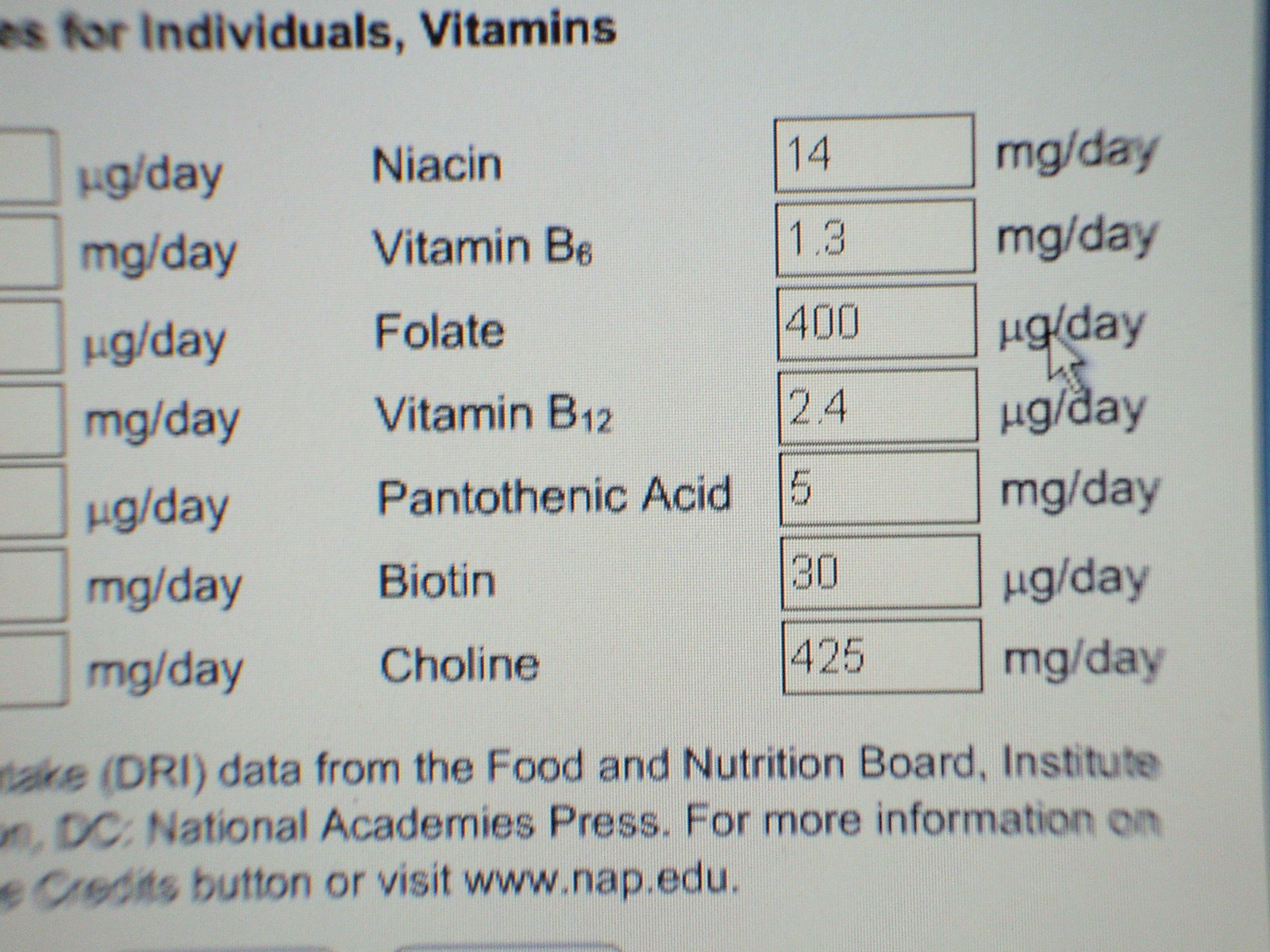This black and white photograph captures a close-up of a computer screen, displaying a form for tracking daily vitamin intake. The screen features a white background with black text, detailing individual nutrient recommendations in vertical, square text boxes. Vitamins such as niacin, vitamin B6, folate, vitamin B12, pantothenic acid, biotin, and choline are listed, each accompanied by their daily recommended dosages: niacin at 14 milligrams, vitamin B6 at 1.3 milligrams, folate at 400 micrograms, vitamin B12 at 2.4 micrograms, pantothenic acid at 5 milligrams, biotin at 30 micrograms, and choline at 425 micrograms. The text, partially cut off on the left side, includes a reference to data from the Food and Nutrition Board Institute, National Academies Press, and a link to www.nep.edu for more information. A mouse cursor is visible on the screen, suggesting ongoing interaction with the form.